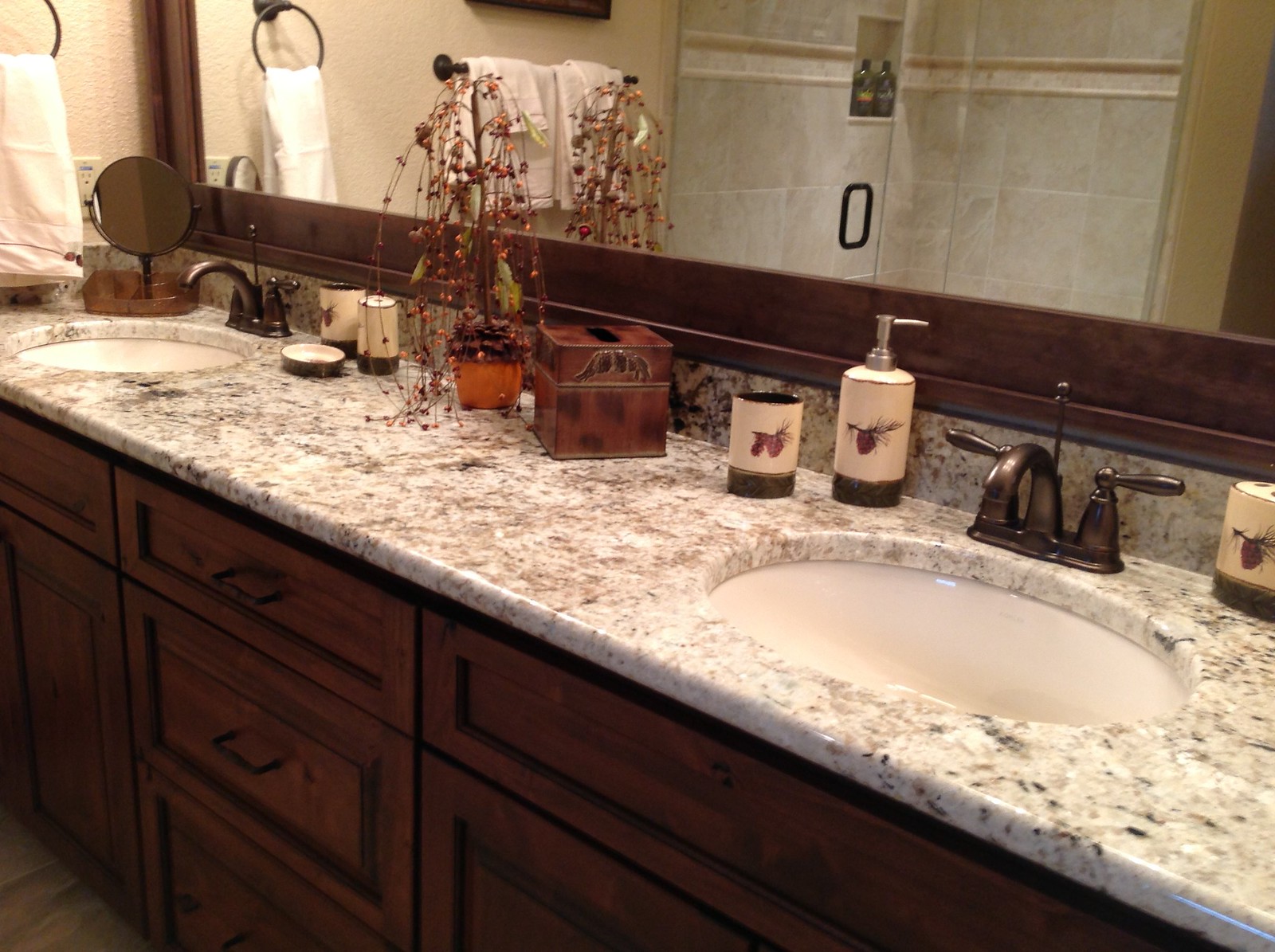The photograph showcases a luxurious double sink setup, likely located in an upscale restaurant or hotel bathroom. The image is captured in portrait orientation. 

In the upper left to the upper right center of the image, a large mirror framed in wood dominates the wall. Reflected in the mirror, you can spot a black towel ring attached to a cream-colored wall, holding a slightly wrinkled towel. Further into the reflected background, another towel holder is visible, laden with several towels, and the suggestion of a shower area with extensive tiling is present. Glass panels cover parts of the shower, with what appears to be shelves holding shampoo and conditioner bottles.

Below the mirror, a long vanity countertop stretches across the wall. On the countertop, against the wall, there is an electrical outlet. Nearby, a circular makeup mirror is set up, adding functionality to the space.

Centered in the image, the double sink features dark metal faucets. Various items are neatly arranged around the sink area: a white ceramic soap dispenser, a white cup possibly meant for holding toothpaste, and a toothbrush holder decorated with tiny circles on its lid. Additionally, there is a plant art piece, likely artificial, and a small bronze box serving as a piece of decorative art.

To the right side of the image, the sink and faucets are shown more clearly, emphasizing the luxurious and stylish elements of the room's design.